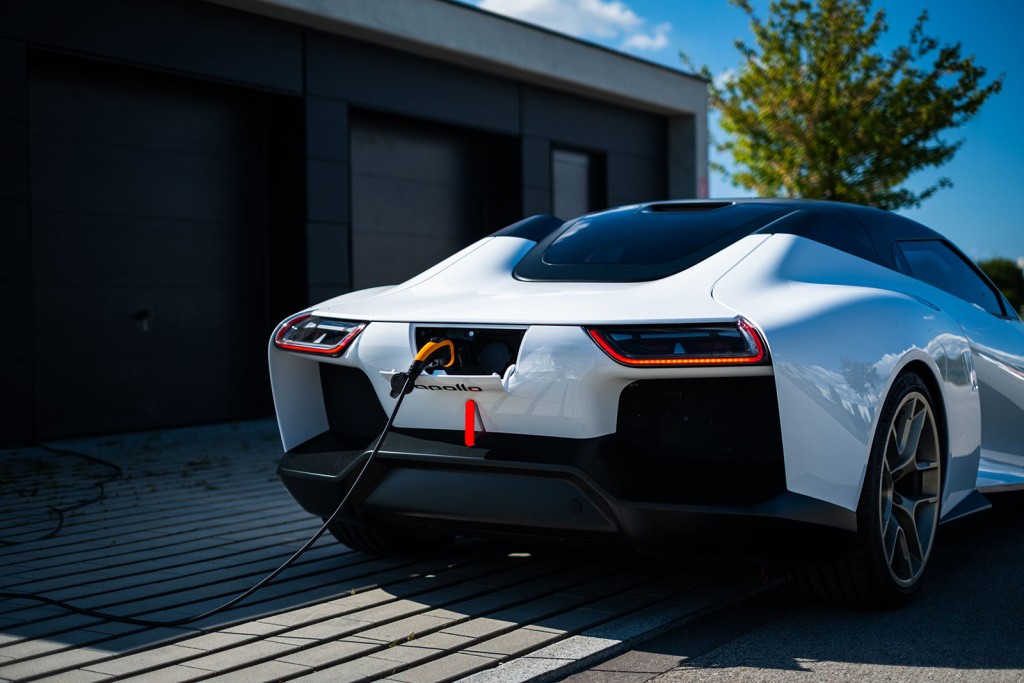The image captures a sleek, modern electric sports car in the process of being charged, viewed from the rear. The car, primarily white with a black roof and curved glass windows, features flat, rectangular taillights that slope towards the center. There are noticeable red details around the taillights and an orange connector piece where the black charging cable enters the car. The brand or model, possibly labeled "Apollo," is located just below the charging port. The car is parked halfway on a tiled platform and halfway on a concrete driveway in front of a small house with a garage. In the background, there is a tree and a beautiful blue sky with clouds. Reflections of mountains can be seen on the right side of the car, adding to the scenic setting.